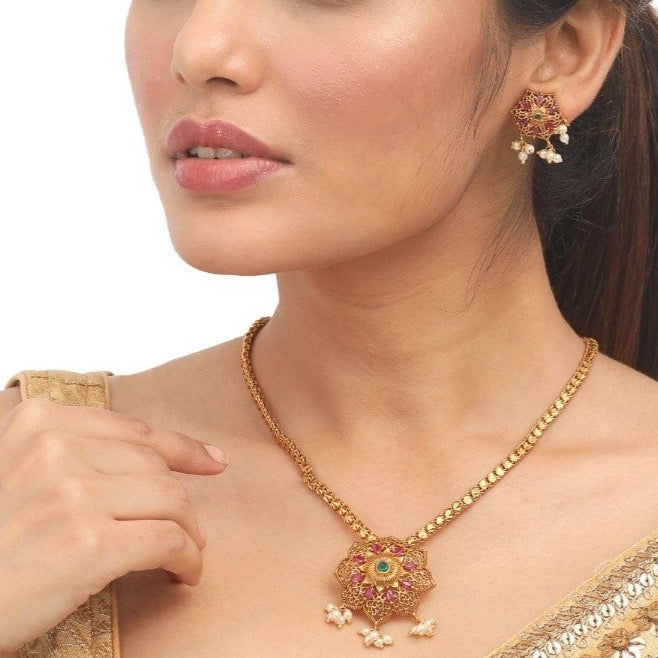The image is an up-close color photograph of a Caucasian woman with fair skin and brown hair pulled back into a ponytail, suggesting a professional photo shoot. The focus is on the elaborate jewelry she is wearing, visible from just below her eyes to slightly under her collarbone. She has her hand delicately held up to her neck, possibly to draw attention to her attire. Her ornate beige dress is off the shoulder, making her intricate necklace the centerpiece of the image.

The necklace features a gold interlocking chain with a prominent, elaborate pendant. The pendant has a striking design: a central green stone set in gold, surrounded by a gold starburst pattern, which is further encircled by a larger red and gold starburst. Hanging from the pendant are three clusters of tiny pearls, each branch-like element holding three pearls. Complementing the necklace, her earrings are designed identically to the pendant but on a smaller scale, replicating the green stone, gold and red starburst, and pearl clusters. Her makeup is skillfully applied, enhancing her overall sophisticated and elegant appearance.